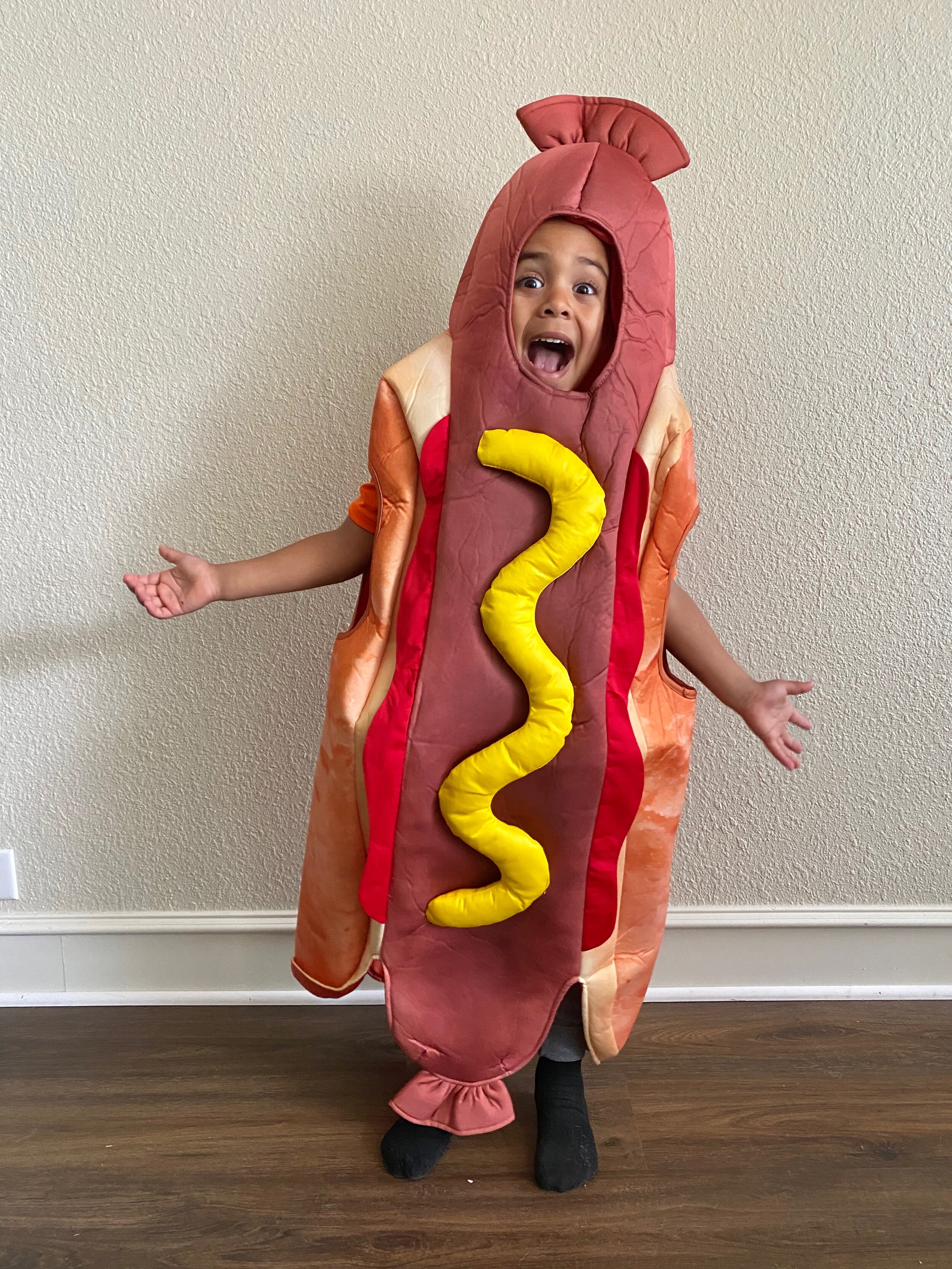This photograph captures the joyous moment of a young African-American child, possibly around five or six years old, dressed in a whimsical hot dog costume. The costume, resembling a frankfurter, envelops the child from head to toe with soft padding, featuring a bun on the sides and a sewn-on yellow cloth strip imitating mustard down the center. The child's face peeks out from a cut-out hole at the top end of the hot dog, radiating happiness. With a wide smile showing their teeth and tongue, the child stands with arms extended, creating an enthusiastic and expansive pose. Their black socks are visible beneath the costume. The setting of the photograph is a home with dark brown wooden floors and off-white walls accented with white baseboards. The overall ambiance captures a lighthearted, festive spirit, with the child clearly enjoying the moment.